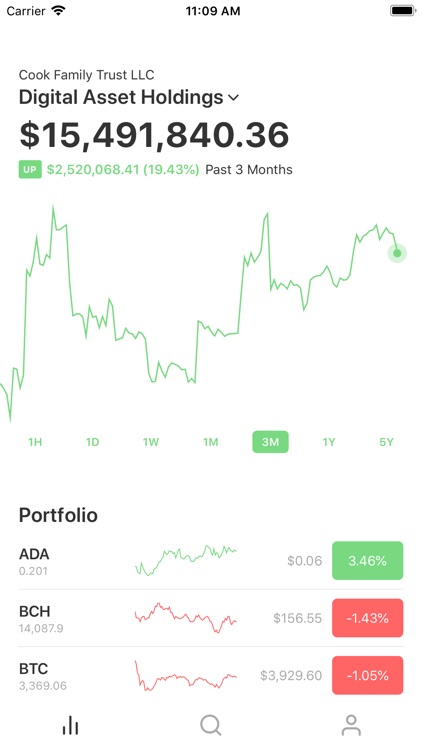The image is a screenshot of a smartphone displaying a financial app with the following details:

- **Top Bar:** A white background with black font indicating the phone carrier, a full Wi-Fi signal icon, the time "11:09 AM" in the middle, and a full battery icon on the right.
- **Header Section:** 
  - Left side: "Cook Family Trust LLC, Digital Asset Holdings" with a downward arrow.
  - Center: A prominently displayed amount of "$15,491,840.36".
  - Right side: A green box with white text stating "UP" and an associated figure "$2,520,068.41" (19.43%), indicating a percentage increase. Beneath this, it states "past three months".
- **Graph Section:** A line chart showing up-and-down trends with a green line ending in a green circle pointing slightly downward.
- **Time Frame:** Below the chart are options for different time frames — 1H (1 Hour), 1D (1 Day), 1W (1 Week), 1M (1 Month), 3M (3 Months highlighted in white text within a green box), 1Y (1 Year), and 5Y (5 Years).
- **Portfolio Section:** 
  - ADA: The portfolio shows an "ADA" entry with a green upward chart and "$0.06" indicating a 3.46% increase.
  - BCH: Below a gray line separating entries, "BCH" shows 14,087.9 units with a red downward line and a gray dollar figure "$156.55". A red box indicates a significant decrease of "minus 143.0%".
  - BTC: Adjacent to "BCH", "BTC" shows 3,369.06 units with a red line trending downward, a gray dollar figure "$3,929.060," and a red box indicating "minus 105%".
- **Bottom Section:** From left to right, there are three ascending white lines, a gray magnifying glass icon (suggesting a search function), and an icon of a person (possibly for a user profile) with round head and shoulders.